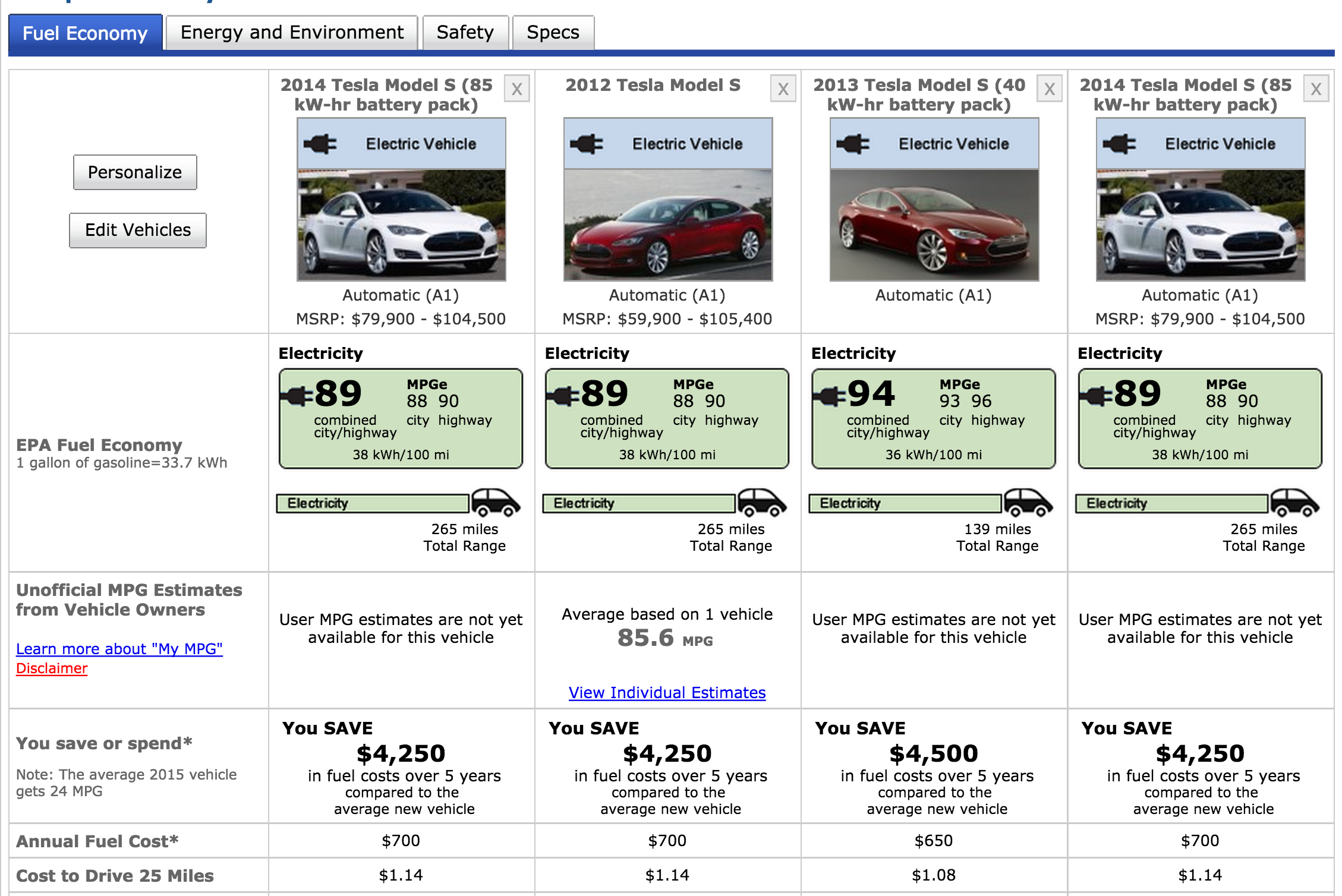Screenshot of a web page displaying a selection of electric cars for sale. The main focus is on four Tesla Model S vehicles, pictured in a horizontal lineup. From left to right, the cars are as follows: 
1. 2014 Tesla Model S with an 85 kWh battery pack,
2. 2012 Tesla Model S,
3. 2013 Tesla Model S with a 40 kWh battery pack,
4. 2014 Tesla Model S with an 85 kWh battery pack.

On the left side of the page, there are options to personalize and edit vehicle information, including EPA fuel economy stats that specify one gallon of gasoline is equivalent to 33.7 kWh. Additional features include unofficial MPG estimates from vehicle owners, a link to learn more about "My MPG," and a disclaimer link. Below these options, there's a section that highlights potential savings or expenditures, noting that the average 2015 vehicle achieves 24 miles per gallon. Furthermore, it provides details on the annual fuel cost and the cost to drive 25 miles.